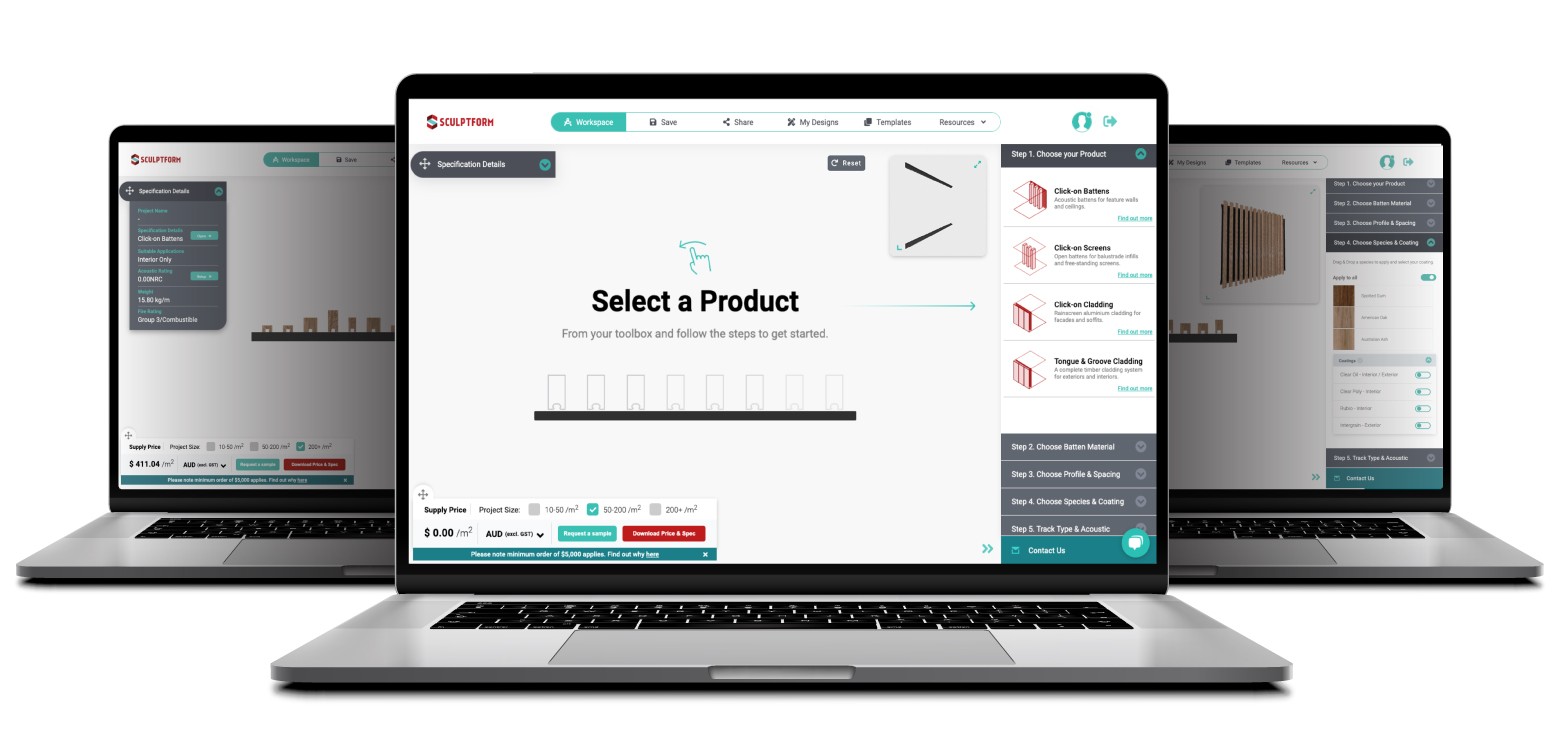A set of three laptops is displayed in the image, each showcasing different versions of the "Sculpt to Form" website. The laptops, all with black keyboards and sleek silver bodies, feature slightly off-silver grid trackpads centrally positioned below the keyboard. The screens predominantly show white backgrounds with sparse black text, presumably displaying web content related to product selections. The content includes details like supply price lines, possibly related to measurements in cubic meters. This detailed depiction captures the essence of multiple stages or variations of the "Sculpt to Form" website.